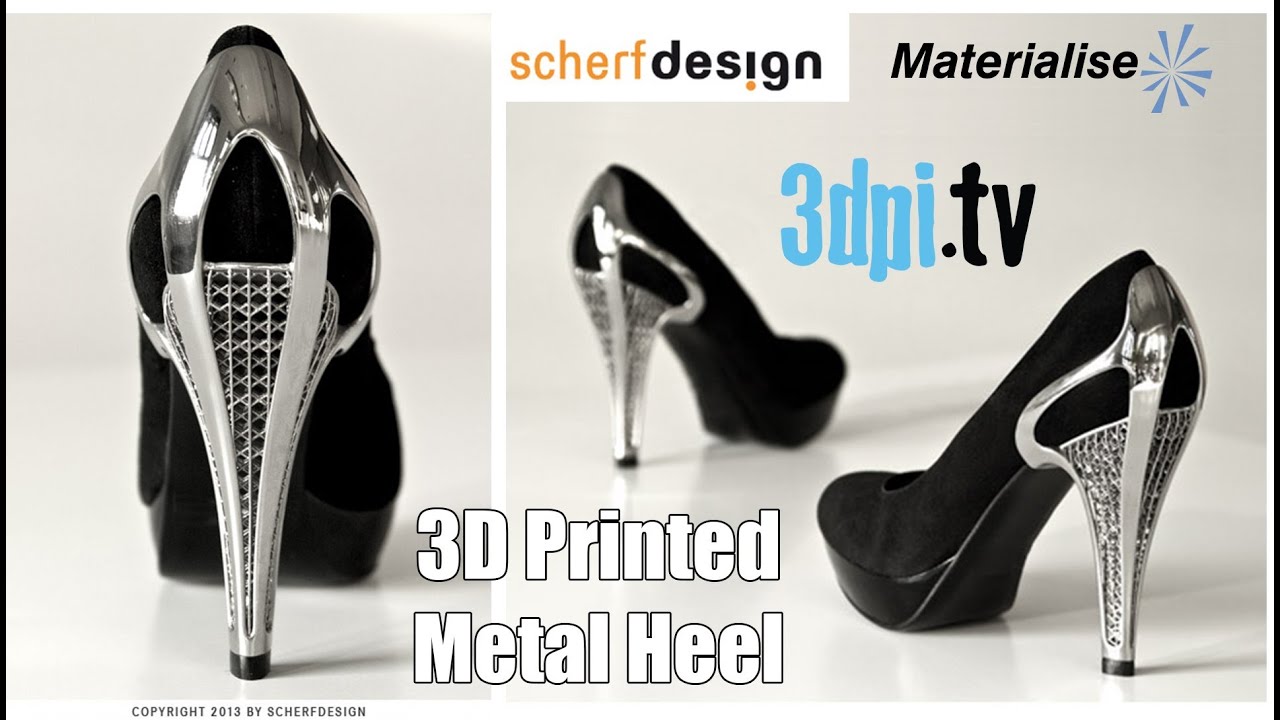The advertisement features an elegant pair of high-heeled black shoes prominently displayed across a split-panel layout. The left third of the ad consists of a vertical rectangular panel with an off-white background, showcasing the sophisticated rear view of one shoe. The heel, reminiscent of a stiletto, drops sharply to a black tip, and is entirely chrome-coated, giving it a sleek and modern appearance. Below this image, the text reads "Copyright 2013 by Scherff Design."

The right two-thirds of the advertisement presents a horizontally oriented layout with two views of the same shoes. The left shoe is slightly out of focus, tilted forward, and angled to the right, whereas the right shoe is in sharp focus, angled to the left, showcasing its chromed heel pointed towards the viewer, with the shoe's tip directed towards the center. This section includes several textual elements: "Scherff Design" and "Materialize" appear prominently, along with a blue circular logo and the phrase "3D printed metal heel" displayed in white at the bottom center. The intricate chrome design of the roughly six-inch heels highlights the innovative 3D-printing technology used, blending high fashion with cutting-edge design methods.